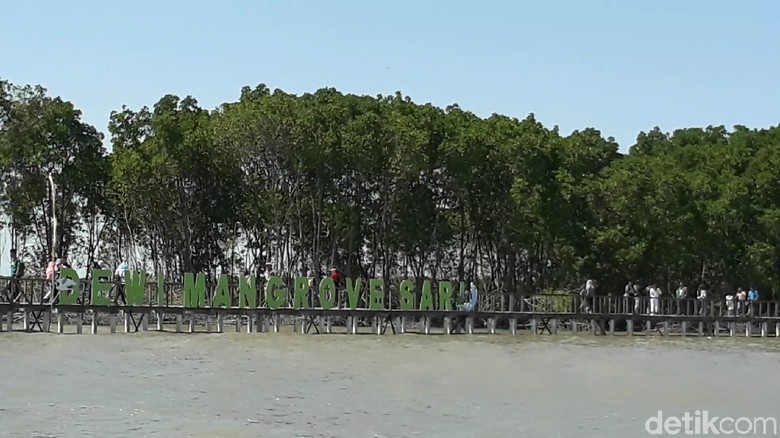The image captures a serene outdoor scene featuring a murky, brownish body of water that dominates the foreground. In the center spans a low bridge teeming with people. This bridge, positioned just above the water, prominently displays large green letters spelling "Dew Mangrove Sar." Behind this structure rises a row of tall trees with slender trunks and lush green foliage at their crowns, stretching from left to right across the image. The clear blue sky forms a striking backdrop above the trees, devoid of any clouds. In the lower right-hand corner, the word "DETICCOM" is visible, adding a mysterious element to the scene. This picturesque setting, possibly within a nature reserve or similar area, captures a blend of human activity and natural beauty.